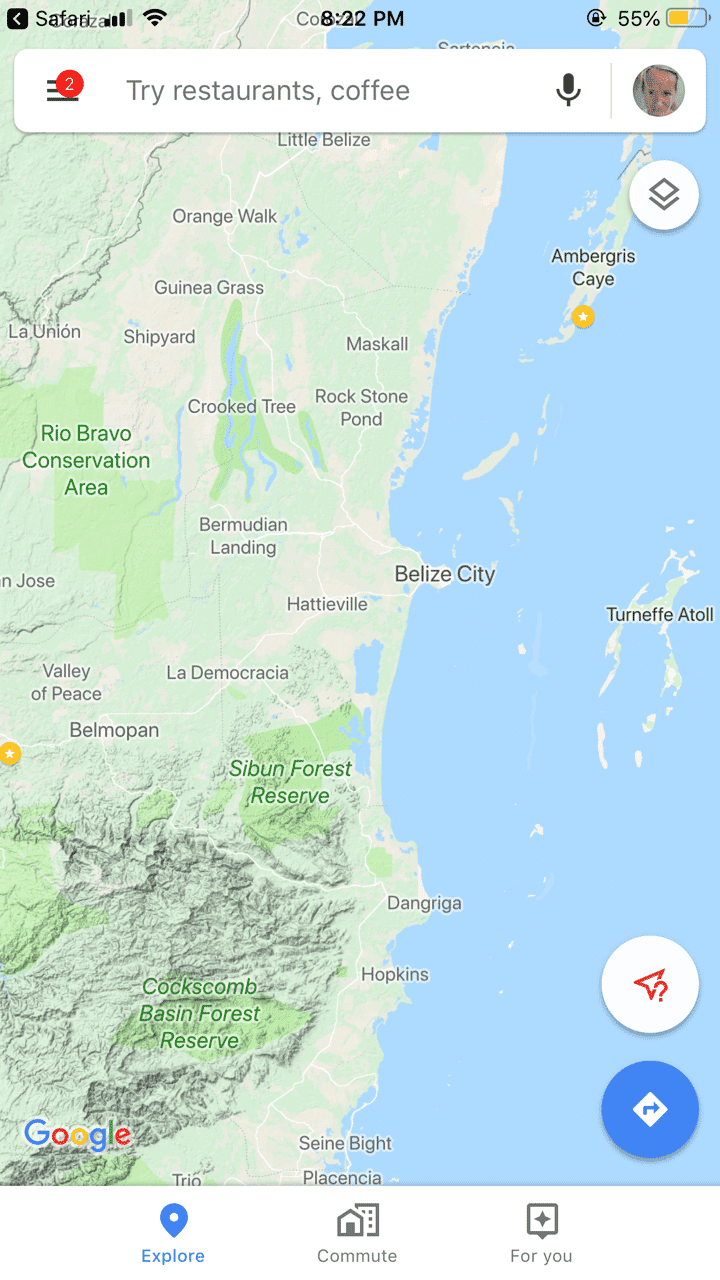This image is a screenshot of Google Maps search results taken on a cell phone in portrait orientation, displaying various interface elements typical of the app. The screenshot, rectangular and much taller than wide, reveals details suggesting it was captured from an iPhone's Safari browser.

At the top left of the image, there's a back arrow inside a black box with the arrow rendered in white, adjacent to the word "Safari." Following this, a network connection status bar reveals a signal strength of 3 out of 4 bars, accompanied by a full Wi-Fi icon. The time reads 8:22 PM. Further along this status bar, a partially obscured icon appears, followed by a battery indicator showing 55% battery life, marked by a yellow meter roughly halfway filled within a horizontally laid battery icon.

Below the status bar, a search bar spans horizontally with a hamburger menu icon, adorned with a red notification bubble displaying the number 2. The suggestions within the search bar prompt, "Try restaurants, coffee," and include a microphone icon on the right, alongside an avatar resembling a man.

In the main section of the screenshot, a map is visible, likely portraying a coastal region as suggested by significant areas of water. The specific area is unidentifiable, hinting at a generic beach town setting. 

At the very bottom of the screen, the familiar Google logo is displayed. To its right, several icons are seen: a blue-highlighted pinpoint for the 'Explore' feature, a 'Commute' icon, and a 'For You' icon, each representing different functionalities within the Google Maps app.